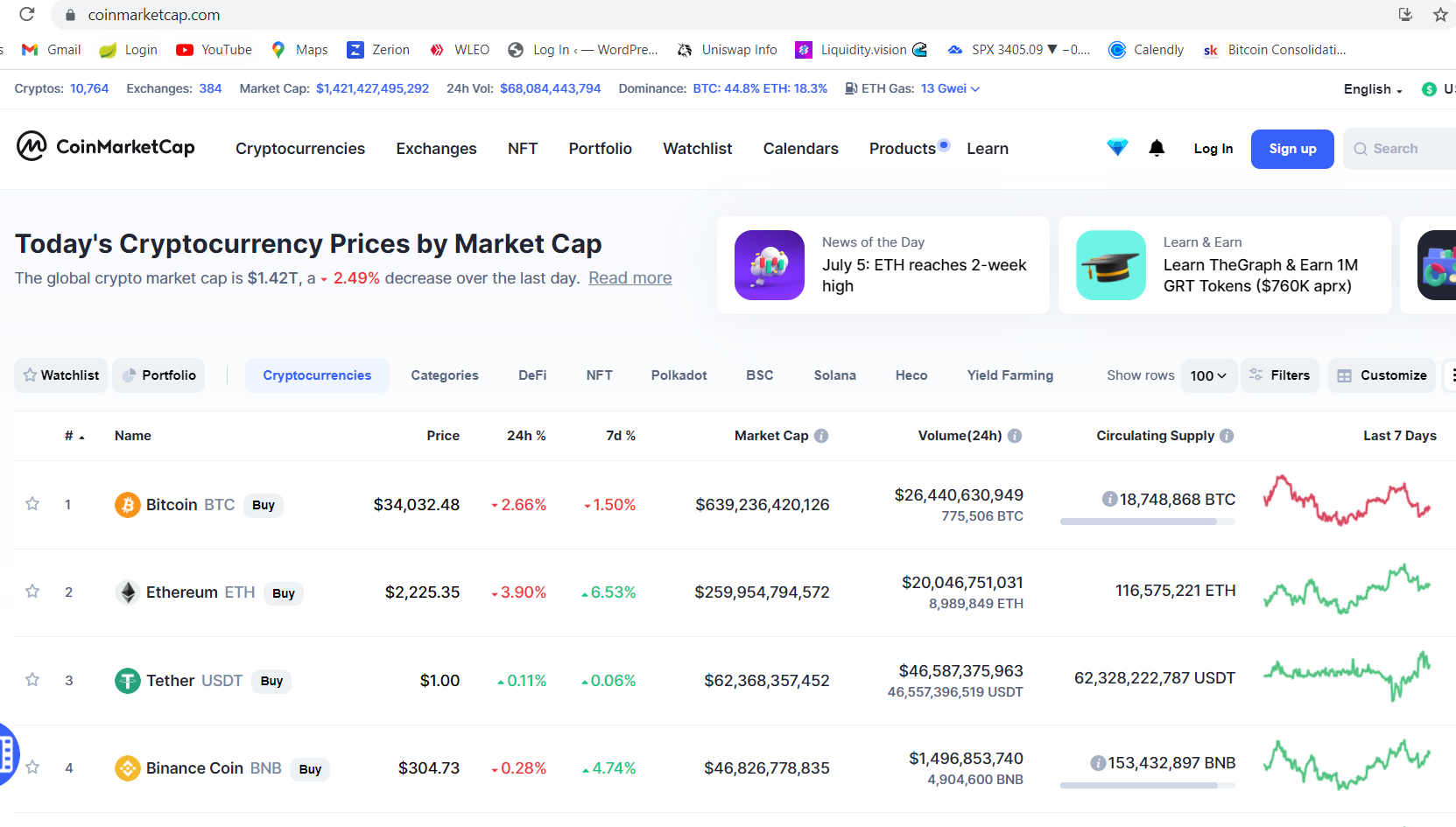This screenshot captures a cluttered computer screen with numerous open tabs visible at the top. Dominating the page is a section featuring an "M" enclosed in a circle. Adjacent to this icon, the text reads "CoinMarketCap" followed by navigation links including "Cryptocurrencies," "Exchanges," "Portfolios," and "Watchlists."

Below this header, the main content showcases today's cryptocurrency prices by market capitalization. A detailed list displays various cryptocurrencies, each accompanied by its respective value. At the far right of each listing, there are dynamic graphs featuring red, green, or blue lines, illustrating market trends.

To the left of these graphs, columns of additional numbers provide further data, including price tags for each cryptocurrency. At the top of the section titled "Cryptocurrency Prices by Market Cap," there are three squares colored purple, light blue, and another color, adding a splash of color to the visual layout.